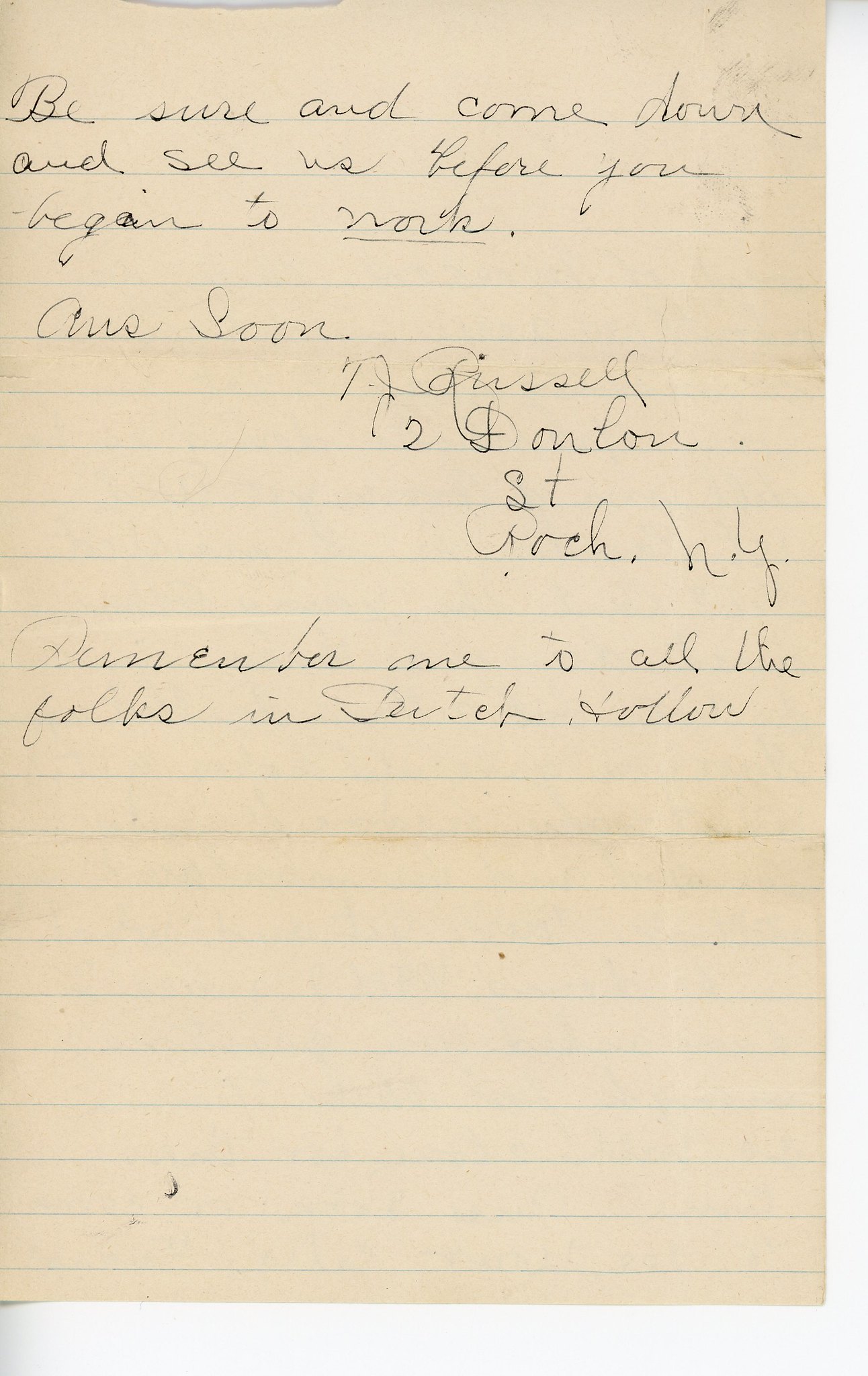The image features a piece of old notepaper with light blue lines, now faded to a light tan or yellowish color, indicating its age. The right side and the bottom of the paper show a distinct white border. Handwritten in cursive with black ink, the note reads, "Be sure and come down and see us before you begin to work." The word "work" is noticeably underlined. Following this, the text becomes increasingly difficult to decipher, but it includes references to an address with "R-O-C-H dot N-Y" and mentions "our soon" and "to all the folks." The handwriting is somewhat messy, contributing to the difficulty in reading the latter parts of the note. The overall appearance and the faded ink suggest that this is a personal, likely farewell, message written to someone who is about to start a new job or endeavor.